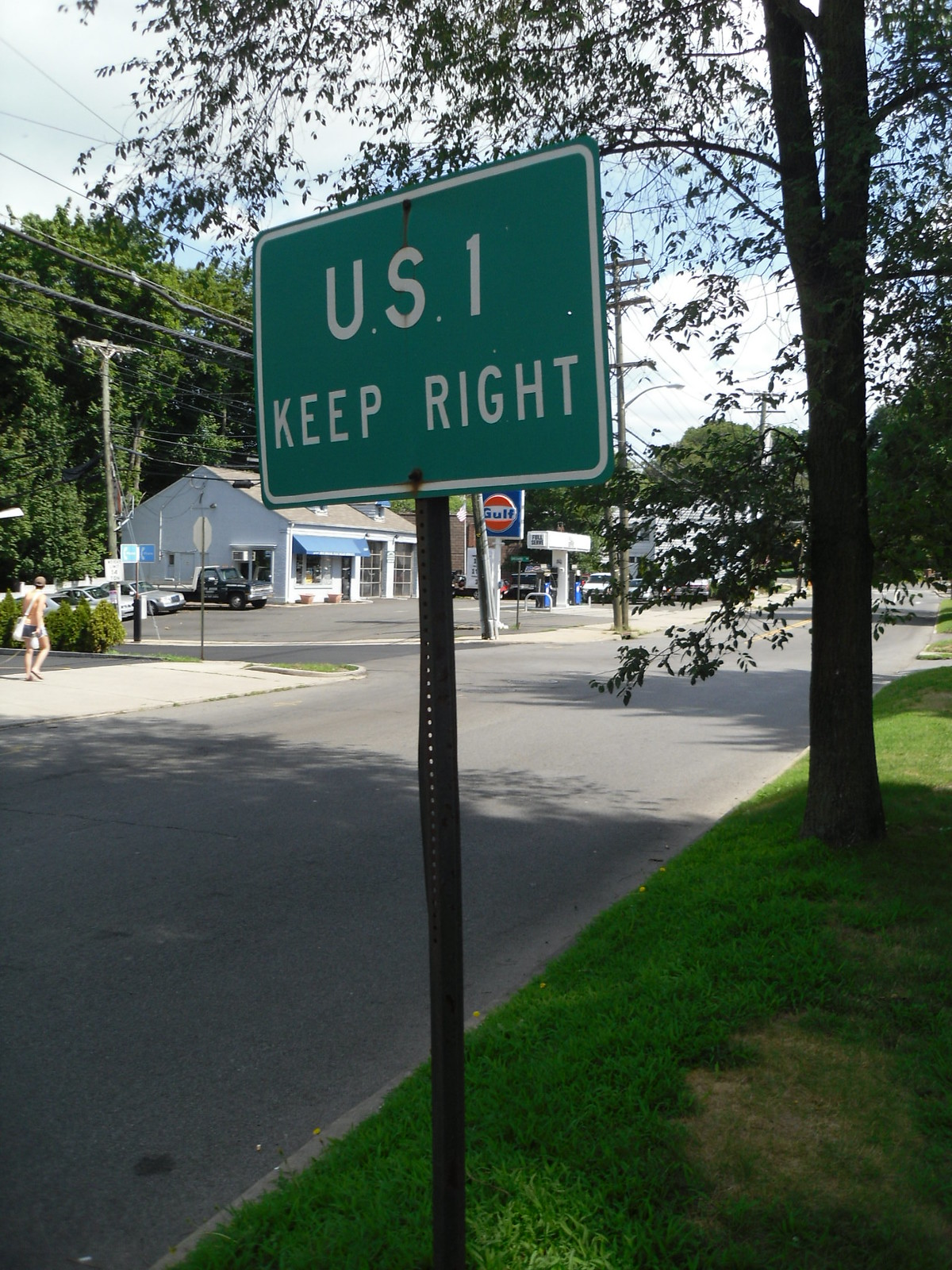In the foreground of this image, a green traffic sign with a white outline and white capital letters reads "U.S. 1, KEEP RIGHT." The sign is mounted on a standard black metal pole with perforated holes, standing in a grassy area adjacent to a light gray asphalt sidewalk. The grass beneath the sign is bright green with some thin patches revealing dirt. To the right of the sign stands a single tree with lush, green foliage. 

In the background, a white building with a blue awning houses a Gulf Gas Station, featuring two gas pumps and a couple of garage doors, hinting at its dual function as a service station. A black pickup truck is parked on the side of the building, while a few other vehicles, partially obscured by bushes, are also visible. 

Further back, tall trees with dense green leaves frame the scene, and a single pedestrian, possibly a female in shorts and a peach t-shirt carrying a white shoulder bag, walks along the far sidewalk. The sky above is mostly overcast with white, fluffy clouds and occasional patches of blue peeking through, casting a soft light over this seemingly tranquil, semi-rural roadside setting.